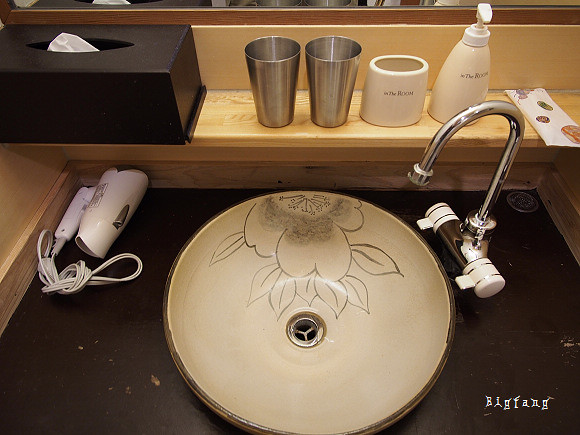The image features a beautifully designed, decorative round sink positioned on a dark brown or black countertop. The sink, resembling a slightly raised bowl, has a pristine white finish accentuated by a light gray line drawing of a partial flower on the upper portion. At the center of the sink is a round drain. To the right of the sink, at around the 2 o'clock position, extends a sleek gooseneck faucet accompanied by two white handles for controlling the hot and cold water.

In the bottom right-hand corner of the image, "Big Fang" is printed in reverse white type. Above the sink sits a functional shelf holding a variety of items: a matching soap pump dispenser and an oval container, likely for toothbrushes, both styled in the same color. Flanking these are two identical metal cups, and to the far right, a sizable rectangular plastic tissue box is present. The uppermost edge of the mirror is visible in the image's frame. In the left-hand corner of the sink, a folded hair dryer has been neatly placed, contributing to the organized yet aesthetically pleasing arrangement.